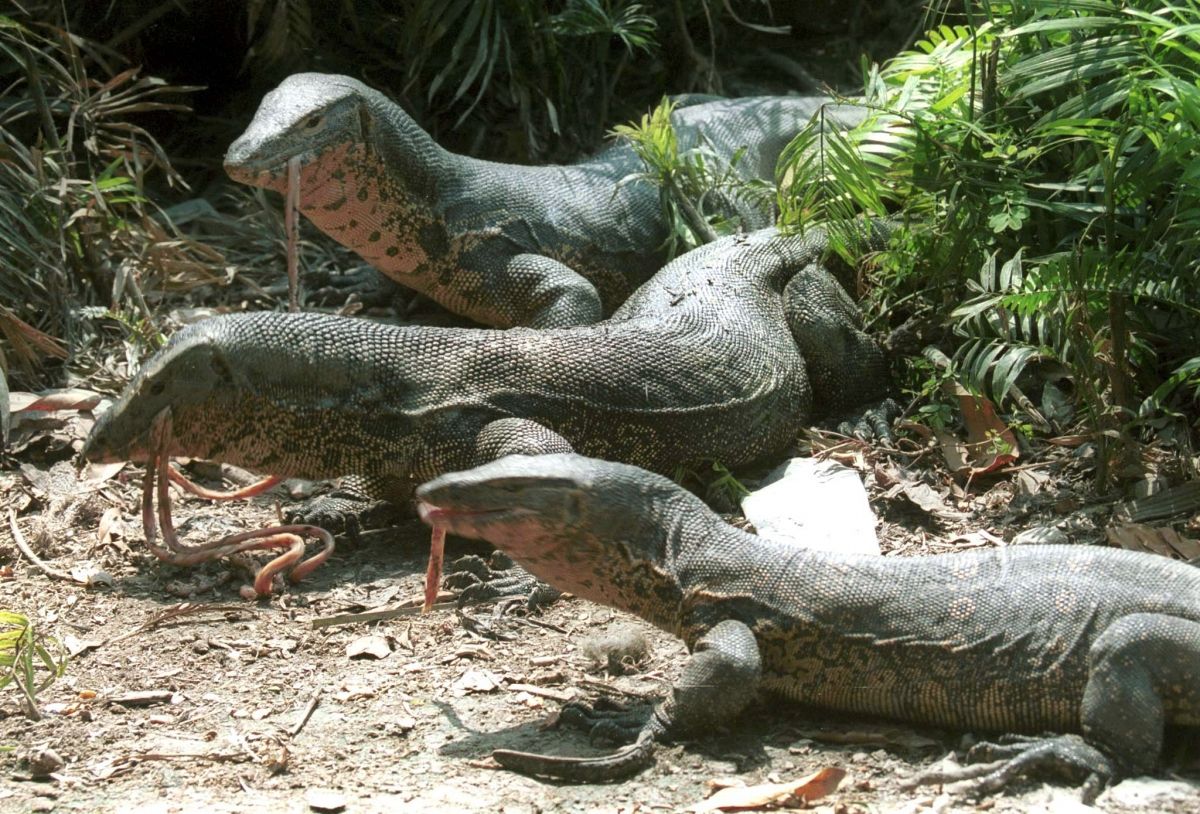In this detailed image, three Komodo dragons, or monitor lizards, can be seen side-by-side with a striking level of detail. Each dragon is holding what appears to be pink intestines in their mouths. The dragons' scales have a reflective quality, showcasing their green tops which transition to a brownish hue underneath. Below their necks, there are distinct pinkish-orange oval patterns blending with the green texture. The rocky, brown terrain they traverse is littered with dead leaves and various plant debris, including branches. Surrounding them are fern-like, green bushes positioned to the left, right, and top center of the photo, with additional smaller plants visible in the bottom left corner. This rich natural habitat sets the stage for these majestic creatures, highlighting their simultaneous primal and picturesque presence.